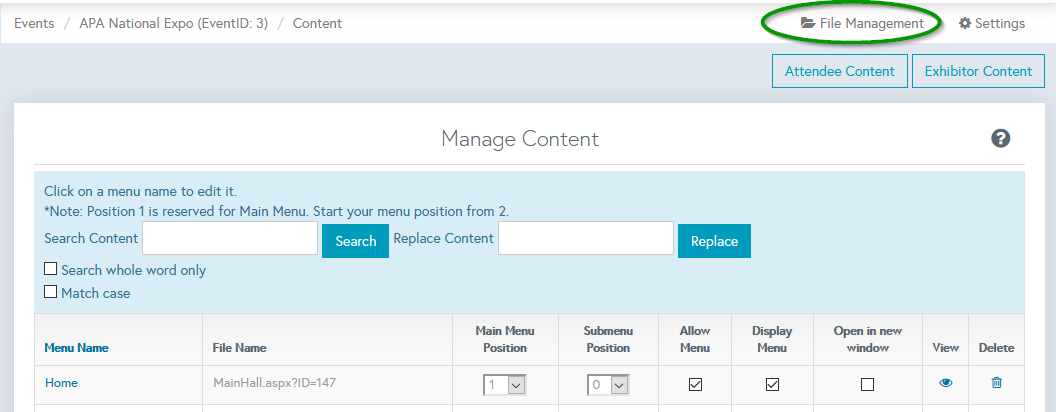This image depicts a software interface for content management, primarily featuring a minimalist color scheme of white, gray, and light blue. At the top of the interface, you'll find navigation headings such as "Events," "APA National Expo," and "Content." A notable section on the right side of the screen is labeled "File Management Settings," with "File Management" distinctly circled in green.

Within a gray horizontal bar, options for "Attendee Content" and "Exhibitor Content" are listed. The central focus of the interface is a light blue box titled "Manage Content," which provides instructions: "Click on a menu name to edit it. Note: position one is reserved for the main menu; start your menu positions from two."

Additionally, there's a "Search Content" section where users can enter terms into a search box, and a "Replace Content" section with a corresponding replace box. Options for "Search Whole Word Only" and "Match Case" can also be selected.

At the bottom of the interface, a gray section features columns headed by "Menu Name," "File Name," "Main Menu," "Submenu," "Allow Menu," "Display Menu," "Open in New Window," "View," and "Delete." Underneath these headers, dropdown menus allow for selecting main and submenu positions. "Allow Menu" and "Display Menu" options are both checked, and the icons for "View" and "Delete" are highlighted in blue, indicating they are active or interactive elements in the interface.